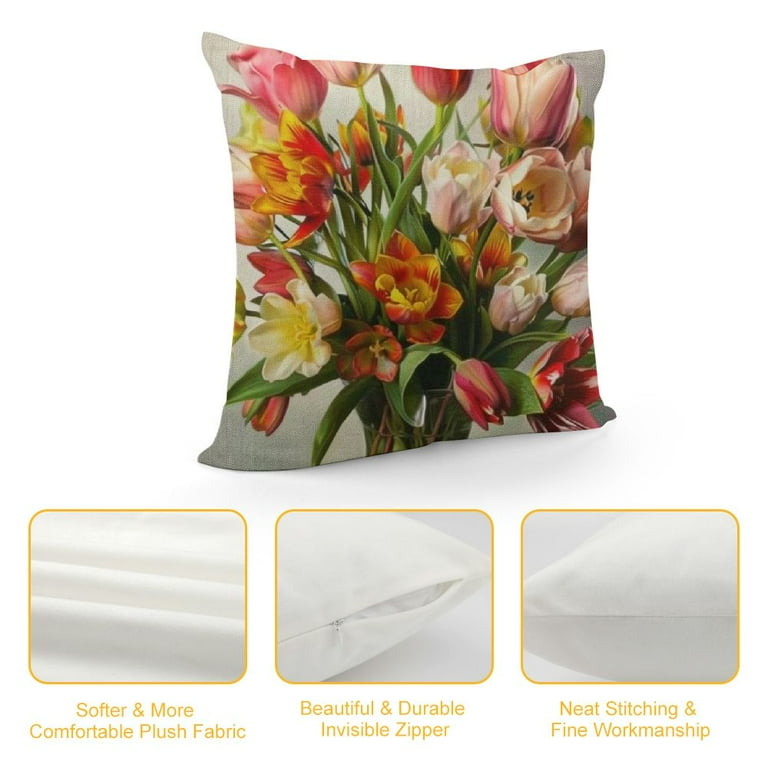This image features a square throw pillow with a predominantly white background adorned with a vibrant bouquet design. The floral print showcases an array of flowers with long green leaves and stems, including pink tulips, white tulips, roses, and a striking red-and-yellow flower with spiky petals. The flowers occupy most of the pillow's surface, with minimal white space, and the top of a glass vase is visible at the bottom, hinting that the bouquet is placed in it.

Beneath the primary image of the pillow, three smaller photos are arranged in a row against a light gray background. The first photo displays a neatly folded piece of soft, plush fabric, labeled "softer and more comfortable plush fabric" in yellow font. The second image shows the pillow with its invisible zipper partially open, revealing some of the inner stuffing, labeled "beautiful and durable invisible zipper." The third image focuses on the pillow's side, highlighting its neat stitching and fine workmanship, with the label "neat stitching and fine workmanship" in the same yellow font.